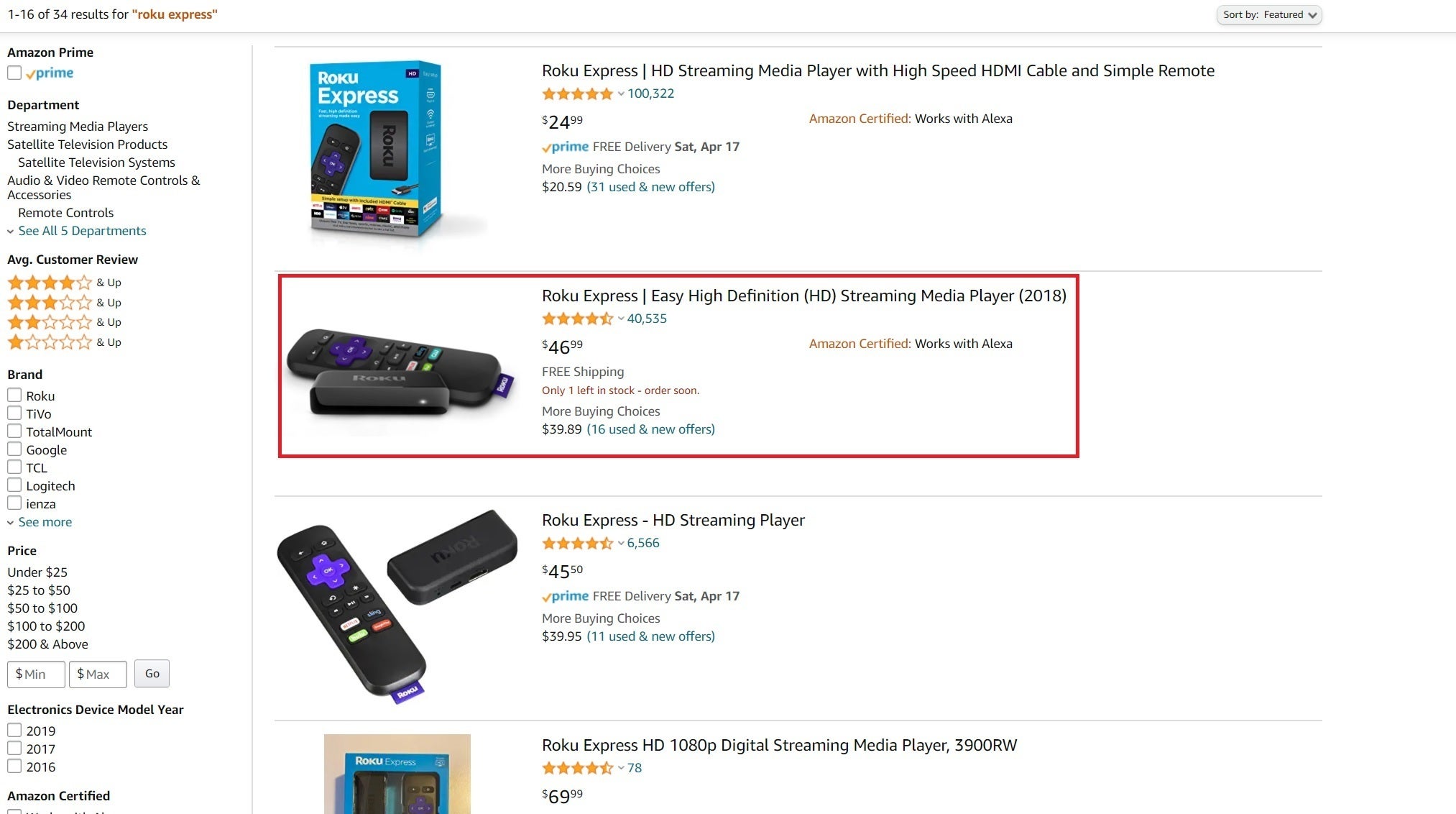**Detailed Caption:**

This image is a screenshot of someone searching for a product on Amazon. On the left side, the traditional Amazon menu is visible. At the top of the menu, "Amazon Prime" is written in bold black text, with an unselected checkbox to the left and the Prime logo to the right. Below this, "Department" is also written in bold black text, followed by several submenu options listed in regular text.

- The first submenu item is "Streaming Media Players."
- The second item is "Satellite Television Products."
- Indented beneath this is "Satellite Television Systems."
- Returning to the main alignment, the next items are "Audio and Video" and "Remote Controls and Accessories."
- Indented under this is "Remote Controls."

Further down, there is an arrowhead pointing downwards with the text "See all 5 Departments" in blue, where "5" is a numeral. Next, in bold black text, it says "Avg. Customer Review" followed by different star rating levels, with options for four out of five stars, three out of five stars, two out of five stars, and one out of five stars.

Following this section, "Brand" is written in bold black text with several checkboxes underneath it. The brands listed are:

- Roku
- TiVo
- TotalMount
- Google
- TCL
- Logitech
- Lenza

Another downward-pointing arrow is beneath these checkboxes, with the text "See more" in blue. None of the checkbox options are selected.

Towards the right side of the image, there is a red rectangular border around a specific product titled "Roku Express." The product description below the title reads "Easy High Definition (HD) Streaming Media Player (2018)," with a black line divider separating the lines.